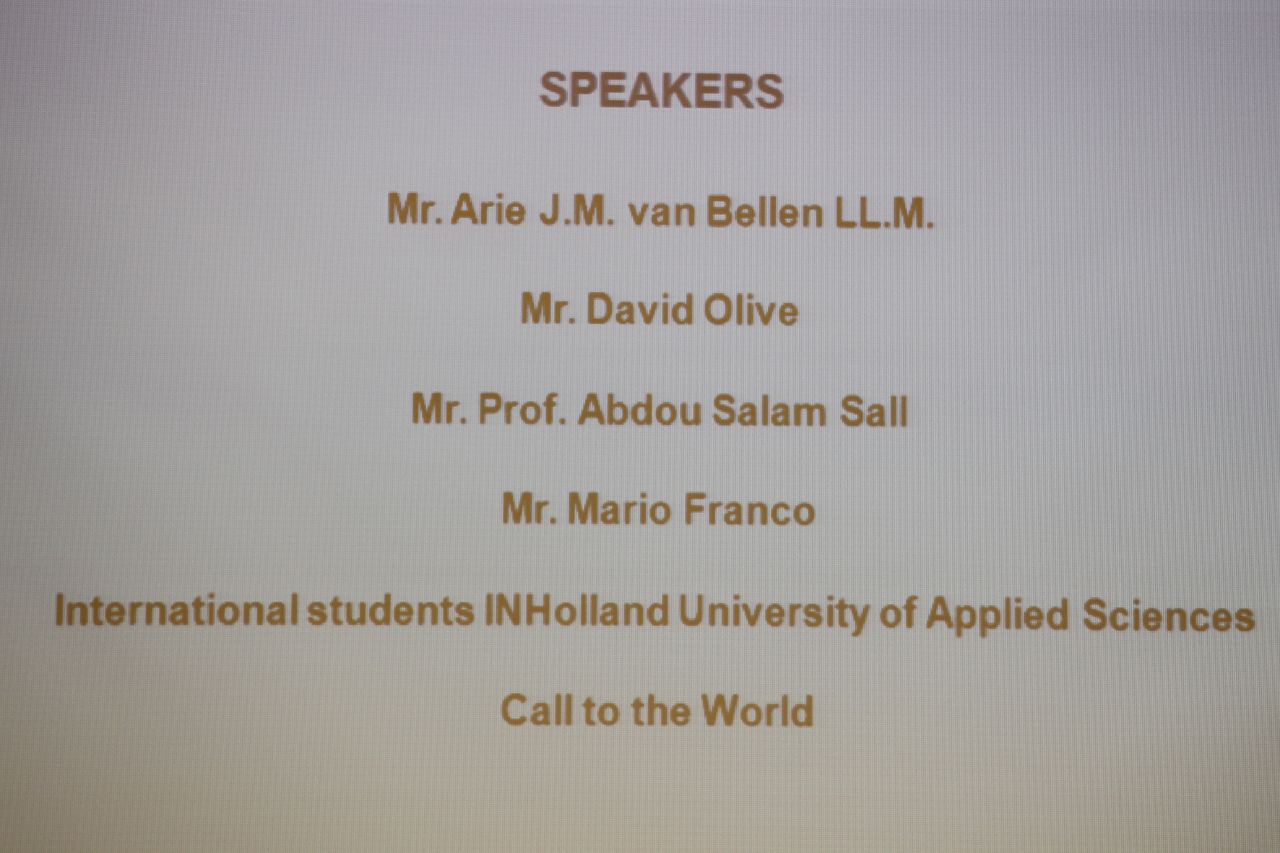The image appears to be a photograph of a computer or projection screen, characterized by the faint lines typical of such photos. The screen displays a slide with a plain white background and centered brown text in two shades. At the top, in all capital letters, is the word "SPEAKERS." Below this heading, the listed speakers are: Mr. Ari J.M. Van Bellen, LL.M., Mr. David Olive, Mr. Professor Abdu Salam Sahl, and Mr. Mario Franco. Following the list of speakers, the text reads, "International students in Holland University of Applied Sciences. Call to the world." The text layout is orderly, with uniform spacing between the names and proper capitalization throughout.